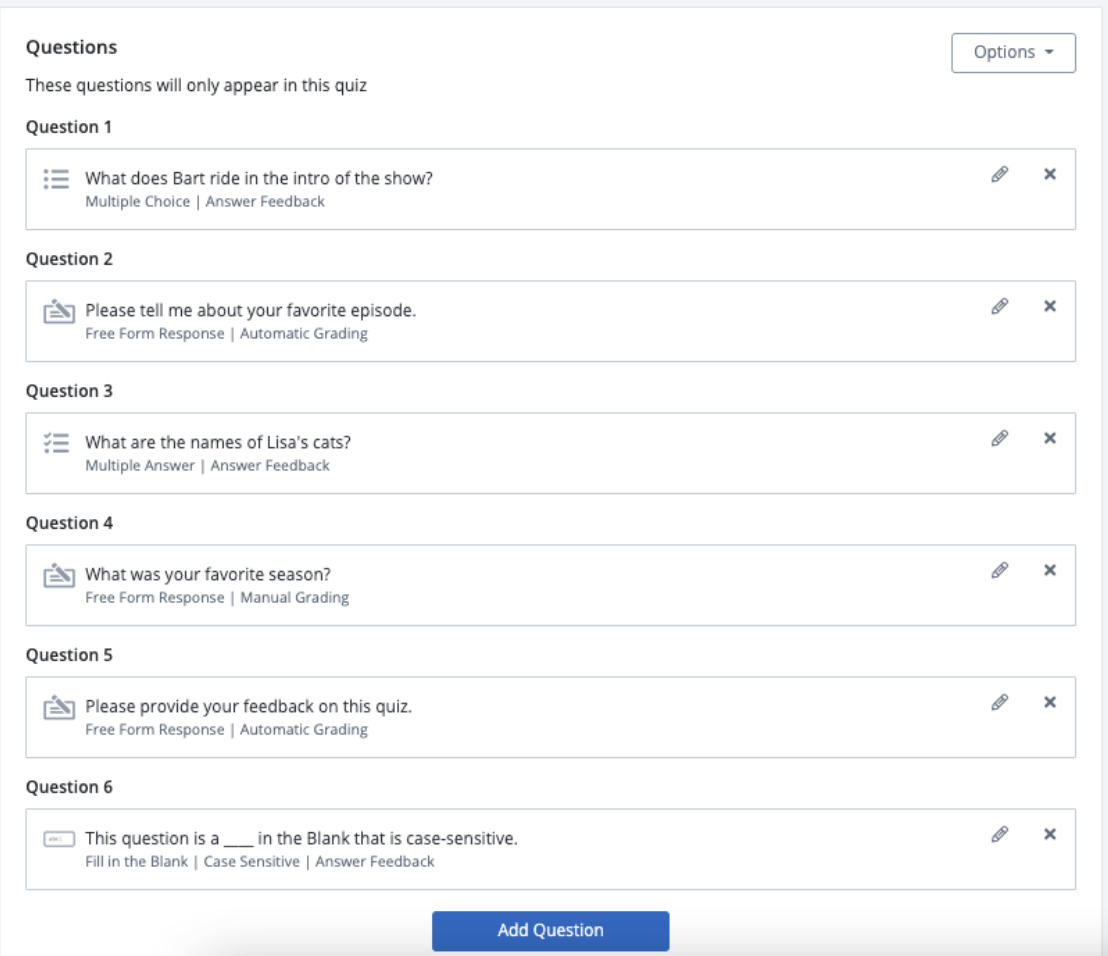**Screenshot of Quiz Page with Questions and Options**

The image captures a detailed quiz interface, starting with a bold heading that reads "Questions." Below this, a subheading states, "These questions will only appear in this quiz."

1. **Question 1:** "What does Bart ride in the intro of the show?" 
   - This is a multiple-choice question, featuring a dropdown button for answer selection. It includes answer feedback and icons of a pencil and an X mark.

2. **Question 2:** "Please tell me about your favorite episode."
   - This is a freeform response question with automatic grading. It is accompanied by a pencil icon and a checkmark.

3. **Question 3:** "What are the names of Lisa's cats?"
   - This is a multiple-answer question with answer feedback. It includes a pencil icon and either a question mark or an X mark at the end of the box.

4. **Question 4:** "What was your favorite season?"
   - This is another freeform response question but with manual grading. Consequently, it has a pencil icon and an X mark at the end.

5. **Question 5:** "Please provide your feedback on this quiz."
   - This is a freeform response question with automatic grading, featuring the usual pencil icon and an X mark.

6. **Question 6:** "This question is a blank in the blank that is case sensitive."
   - This query requires a fill-in-the-blank response, emphasizing case sensitivity. It comes with answer feedback and the pencil and X icons.

At the bottom of the page, there is an option labeled "Add Question," suggesting the ability to include more questions to the quiz.